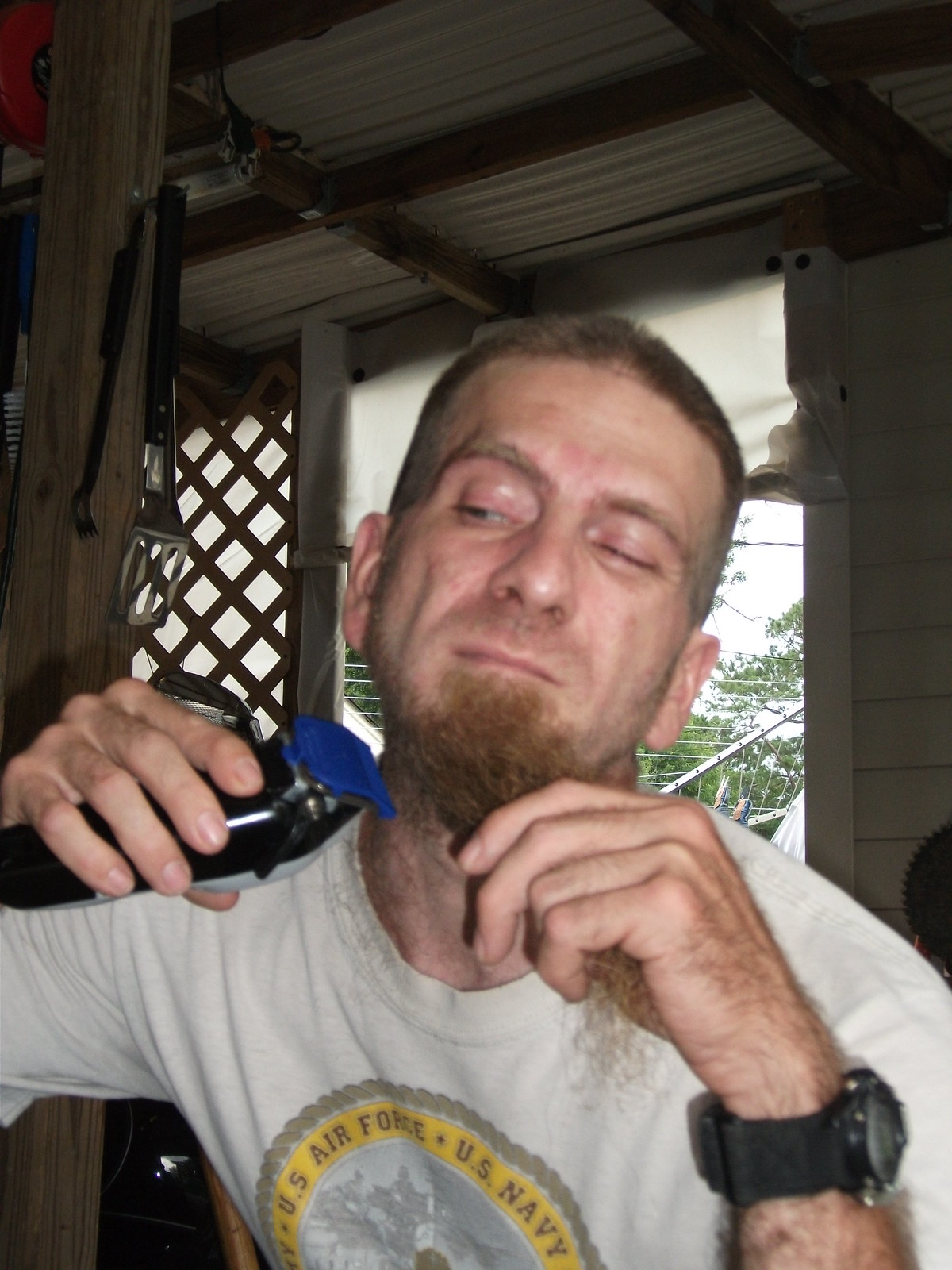A middle-aged man with fair skin and short brown hair is meticulously grooming his long, reddish-brown beard. He holds the beard away from his face with his right hand, which sports a thick black wristwatch. In his left hand, he grips a black electric shaver equipped with a blue guard, approaching his face as he focuses downward on the task. Dressed in a white, short-sleeved t-shirt featuring a military graphic in a circular pattern that includes the U.S. Air Force and U.S. Navy, he stands in an indoor setting with natural elements visible in the background. Through an open door behind him, a clothesline, trees, and a blue sky are discernible, indicating he is likely on a porch or in a garage. The indoor backdrop includes a lattice panel, house siding, and a metal roof supported by wooden framing. The image, taken in portrait format and color, captures the man in the act of refining his beard, pulling it taut as he shaves, giving the viewer a delicate glimpse of his personal grooming routine.